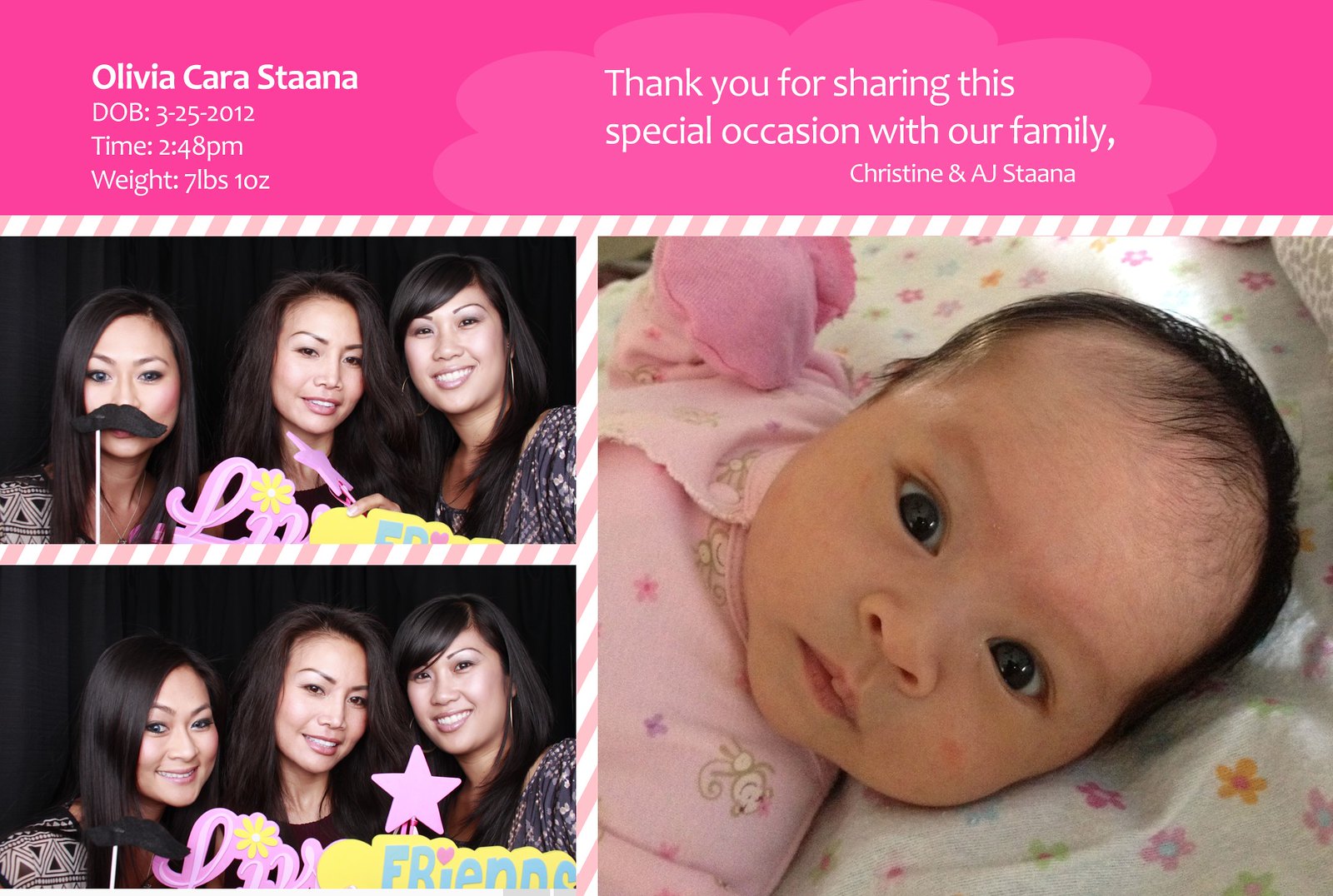The image is a heartfelt thank you card, seemingly for a child's birth or naming celebration. Dominating the top of the card is a large pink bar, displaying the birth details: "Olivia Cara Stanner, D.O.B. 25th March 2012, time 2.48 p.m., weight 7 pounds 10 ounces." Just below, a message reads, "Thank you for sharing this special occasion with our family, Christine and AJ Stanner."

On the left side of the card, two photos feature three middle-aged women, possibly of Asian descent, all with black hair, posing with playful photo props—like a stick-held mustache and a wand with a star. These photographs capture the joyous, celebratory spirit of the occasion. Meanwhile, the right side of the card is adorned with an image of a baby girl dressed in a pink dress and mitts, lying on a white floral blanket. The overall layout captures both the announcement of Olivia's birth and the joy shared among family and friends.